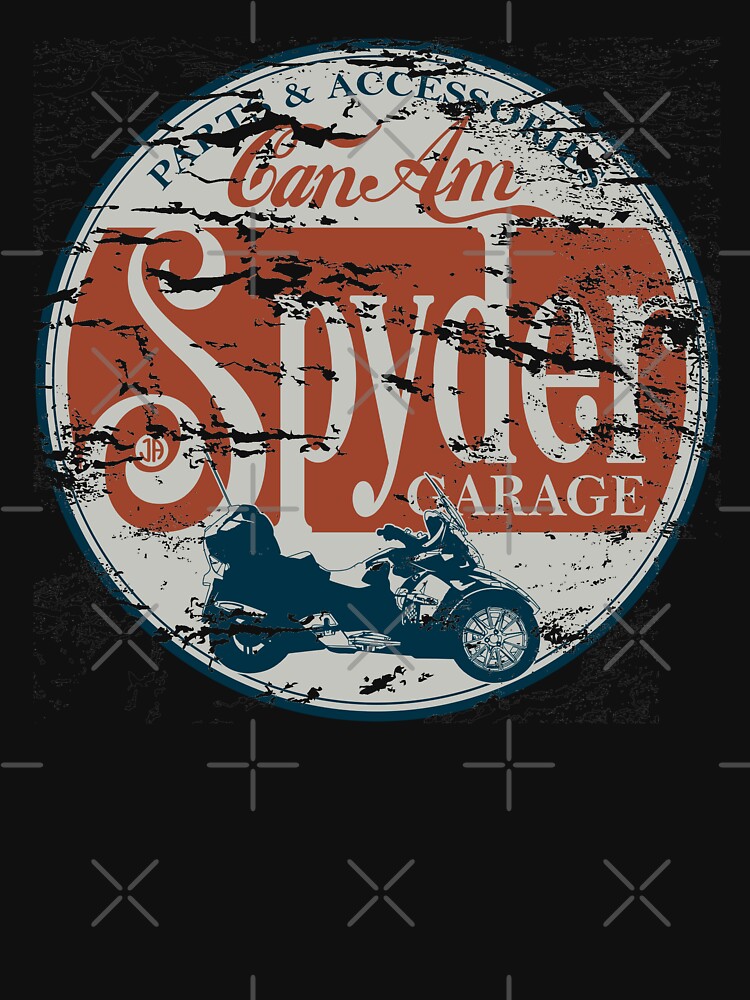This detailed image features a large, rectangular retro-style metal sign reminiscent of those found in old garages, showcasing an emblem with an intentionally distressed and weathered look. The sign prominently displays a bold red banner in the center with elegant white lettering that reads "SPYDER GARAGE" (S-P-Y-D-E-R G-A-R-A-G-E). Above this banner, the name "CAN-AM" is presented in striking red letters. Crowning the top of the emblem, the words "Parts and Accessories" are arched in blue letters. The bottom part of the emblem features a vintage motorcycle positioned against a white background, depicted in black and blue hues, indicating it as an older model. The overall emblem and text bear Coca-Cola style font and color choices, contributing to the nostalgic feel. The sign's weathered appearance includes intentional scratches and black marks, suggesting either a marred paint surface or an artistic choice to simulate age. The background of the image itself is black and overlaid with visible light gray X marks and crosses, indicating it is a stock photo.